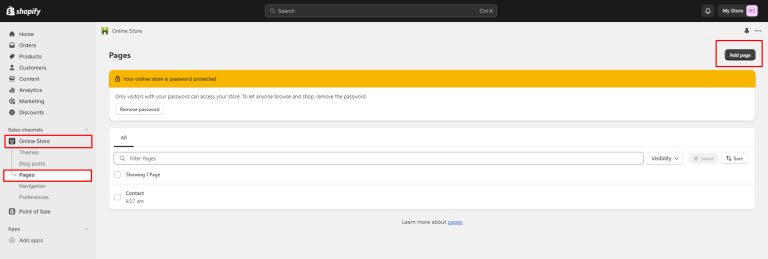This image is a screenshot of a Shopify website displayed on a computer screen. At the very top, a black horizontal navigation bar stretches across the entire width of the screen. On the left side of this bar, there is a white Shopify logo consisting of a shopping bag with a dollar symbol inside it, followed by the text "Shopify." In the center of the bar is a search bar, while on the far right, there's a link that says "My Store."

Below the black navigation bar, the interface is divided into two main sections. On the left, a vertical gray sidebar features a menu of different categories listed in white text. These categories include, from top to bottom: Home, Orders, Products, Content, Analytics, Marketing, and Discounts. Within this sidebar, "Online Store" is highlighted with a red rectangle around it, indicating it has been selected. Further down, "Pages" is also highlighted with a similar red rectangle around it.

The main content area to the right of the sidebar is mostly a large white rectangle, which occupies the majority of the screen. Near the top of this white section, there is a yellow notification bar that spans horizontally across the image about two-thirds of the way up the screen. The message in this yellow bar states, "Your Online Store is password protected."

Further down within the main white area, there are several elements, including a "Filter Pages" box and various other options, though they are less prominently displayed and not central to the screenshot's focus.

Overall, the screenshot captures the administrative interface of a Shopify website where the user is managing their online store, specifically focusing on the Pages section within the Online Store category.